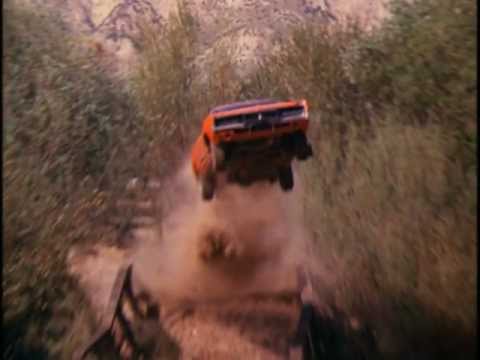In this dynamic image, we see an iconic scene reminiscent of the Dukes of Hazzard, featuring an orange car, likely the General Lee, mid-air, showcasing a thrilling jump. This classic car, which might be a Dodge Charger rather than a Pontiac GTO, captivates attention with its black grill prominently visible. The car is centered in the image, its front end lifted higher than the rear, giving the impression of an upward, angled leap. 

Below the car, a substantial cloud of dirt billows up, indicating a high-speed takeoff from a dirt path, possibly leading over a wooden bridge. This bridge is flanked by fences visible towards the bottom edges of the image. Surrounding the scene is a lush landscape filled with green trees and underbrush, creating a stark contrast to the brown dirt and the vibrant orange of the car. In the background, a rock wall or hills devoid of much vegetation peek through the greenery, adding depth to the outdoor setting. The car's four black wheels and the underside are clearly visible, emphasizing the height and intensity of the jump.